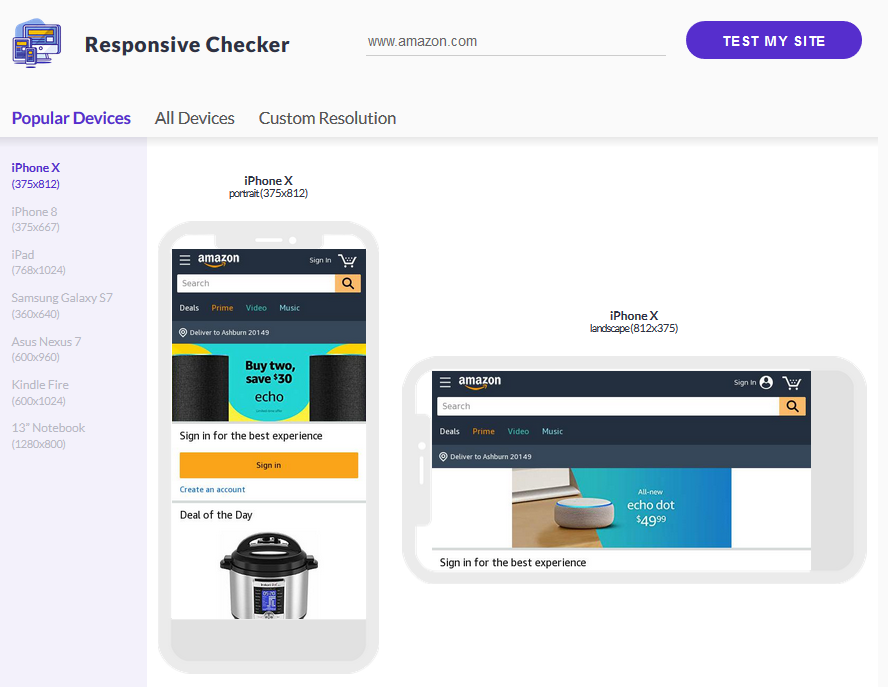The image depicts a website tool known as a "Responsive Checker." This tool is utilized to verify the responsiveness of a website across various devices and resolutions. The background of the image is predominantly white with subtle shades of light gray.

At the very top of the screen, on the left-hand side, is the title "Responsive Checker" accompanied by a small icon adjacent to the text. Below this, there is a search bar containing the URL "www.amazon.com." Next to the search bar is a prominent purple button labeled "Test My Site."

Beneath the search bar, to the left, are three selection options: "Popular Devices," "All Devices," and "Custom Resolution." The "Popular Devices" option is highlighted in purple and has an open menu listing several devices. These devices include the iPhone X, iPhone 8, iPad, Samsung Galaxy S7, Asus Nexus 7, Kindle Fire, and a 13-inch notebook, with each device's screen resolution provided underneath its name.

Adjacent to this menu, occupying a much larger section of the screen, is a display of the iPhone X in both portrait and landscape modes. This section visually demonstrates how the Amazon website appears on the iPhone X in both orientations. The background of this larger display window is white, maintaining the overall clean and minimalistic design of the tool interface.